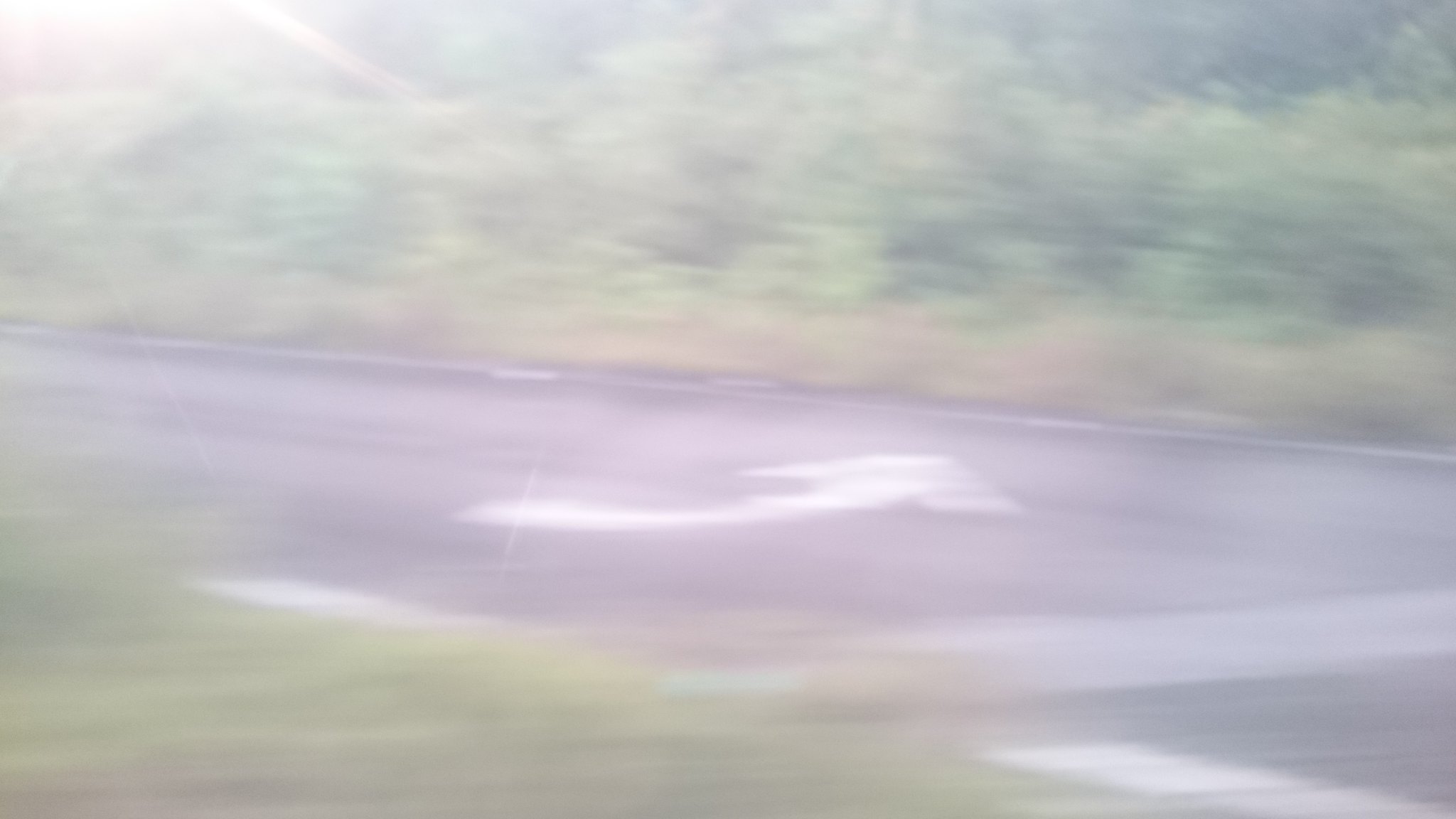A sunlit driveway curves to the right, marked by a prominent white arrow painted on the pavement. To the right of the driveway, there's a lush green landscape adorned with tall trees that create a rich, verdant backdrop. Patches of grass intersperse the bottom left corner of the image, adding texture to the foreground. The top left is illuminated by the soft, golden light of the sun, casting gentle shadows across the scene.